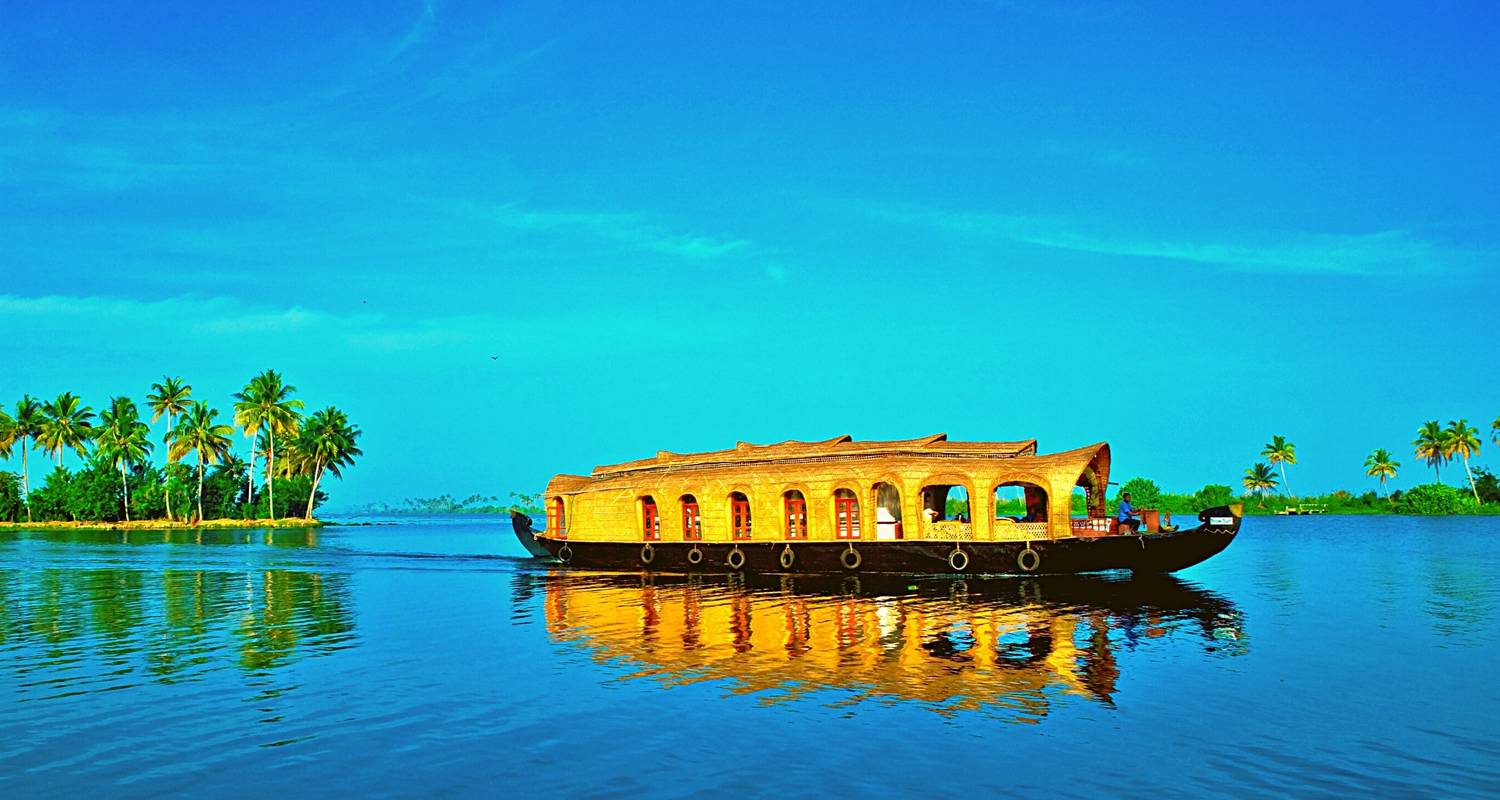In this horizontally aligned, rectangular photograph, an orange boat with a dark wooden bottom glides across calm, vivid blue water that mirrors the vibrant sky above. The scene is set on a bright, sunny day under a clear sky accented with wispy, feathery white clouds. Sunlight glints off the boat, intensifying its orange hue and casting reflections on the tranquil water. The boat's covered sections feature windows with little red coverings and gold circles hanging along the sides. A person in a blue shirt is visible at the uncovered front of the boat, seemingly steering it from a reddish desk. Surrounding the boat are small islands adorned with lush palm trees and green bushes. The scenery conveys a serene and picturesque tropical setting, enhanced by the heightened contrast that makes the vibrant colors pop.